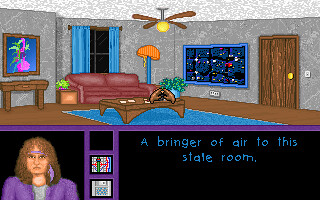The image appears to be an animation, possibly from a video game or a basic TV show. The top half of the image depicts a cartoon living room with dark grey walls, a light grey or white ceiling, and brown wooden floors. The room is furnished with a red couch positioned against the backdrop of two windows. A brown door is visible on the right side of the room, and a large blue rectangular rug lies in the center. In the bottom half of the image, set against a black background, is a light-skinned cartoon woman with long, curly blonde hair. She appears on the bottom left, dressed in a purple suit. To her right, in blue text, the caption reads, "A bringer of air to this stale room."